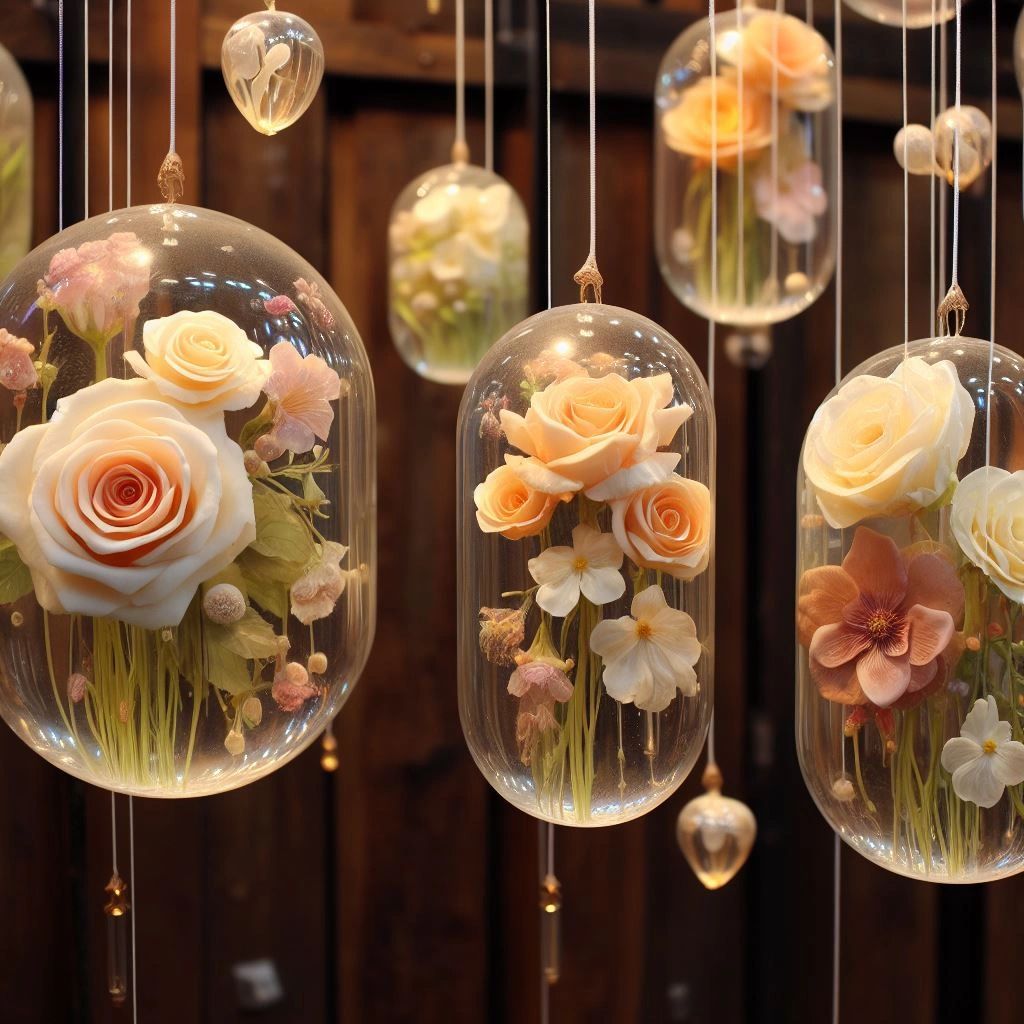The image features a captivating art display of delicate, blown glass orbs and teardrops, each meticulously encasing small bouquets of preserved flowers. These glass orbs and teardrops, primarily oval-shaped but some teardrop-shaped, hang gracefully by transparent threads from what appears to be a wooden ceiling or backdrop. Featured prominently in the photograph are three distinct glass orbs. The leftmost and largest orb contains a striking arrangement centered around a pink rose, accompanied by several smaller roses and decorative white flowers. The middle orb houses a smaller bouquet with a larger pink rose, flanked by two smaller pink roses and two white flowers. The rightmost orb displays a mix of white roses and a pink daisy-like flower. Light entering from the top right illuminates the scene, casting a delicate glow on the preserved flowers and highlighting their soft colors, predominantly white, pink, and beige, with green stems and leaves adding a fresh touch. In the background, partially obscured orbs suggest continuity beyond the frame, enhancing the artistic and ethereal quality of the display.